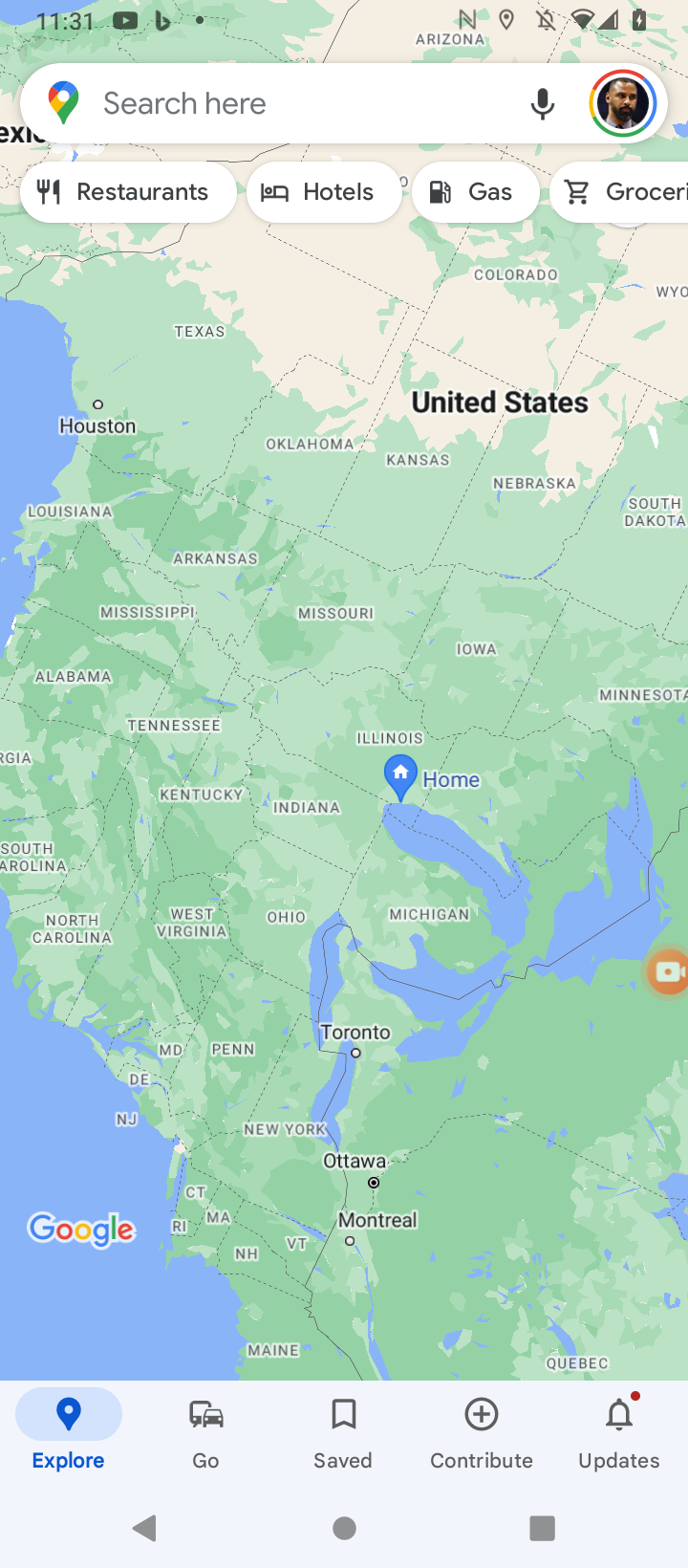This image is a screenshot from a phone displaying a Google Maps view of the United States with a prominent "Home" location marked in Illinois by a blue map pin. The phone interface is visible at the top, showing time (11:31), battery, and connectivity icons. Below this, a Google search bar adorned with the familiar red, yellow, blue, and green colors includes a microphone icon and a profile picture of a dark-skinned man with a beard wearing a suit. The search bar sits above tabs for restaurants, hotels, gas, and groceries, each with black icons. The map is tilted at an odd angle, displaying regions from South Carolina to Minnesota and stretching from part of Canada (including Toronto, Ottawa, and Montreal) down to about a third of Mexico. The lower part of the screen includes navigation options like explore, go, saved, contribute, and updates. The screen hints at open applications positioned near the bottom, including a left arrow in a circle and a small square.